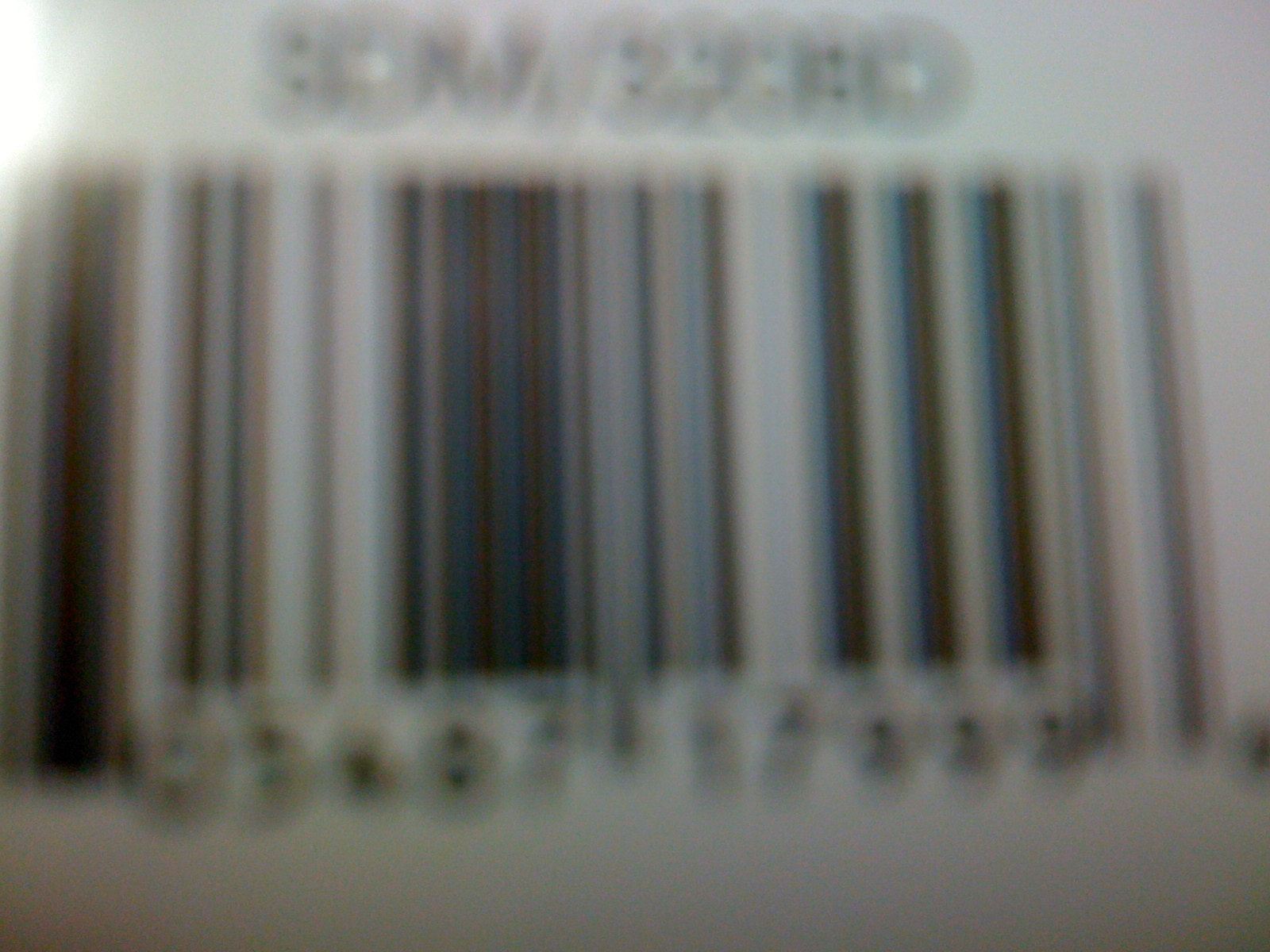The photograph shows a highly blurry and extremely close-up image of a barcode against a white background. The black barcode lines and accompanying text take up most of the frame, but due to the poor focus, no numbers or letters can be clearly discerned. At the top of the barcode, there appears to be a word or a series of characters—possibly "BOWIEOOD"—though the heavy blur renders it virtually illegible. The overall lack of clarity makes it impossible to make out any specific details of the barcode or the text above it.